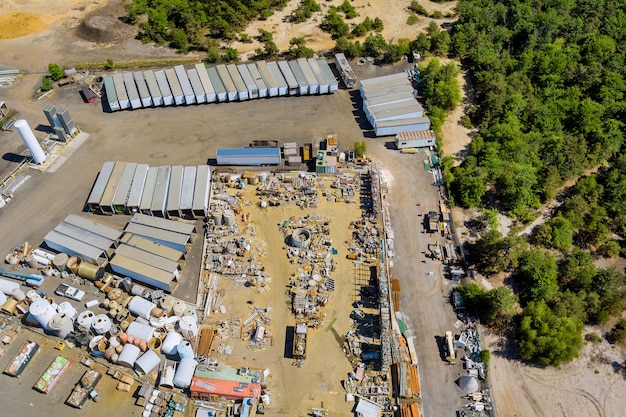This daytime aerial view captures an expansive industrial junkyard and storage facility. At the center of the image is a vast area littered with various machine parts, empty barrels, tanks, and blue containers, all positioned haphazardly in what seems to be a dirt or sand lot. Flanking the left side of the facility, one can see an array of tall tanks resembling silos, while the right side and upper portions of the image are bordered by dense clusters of trees. Alongside the perimeter, particularly the back, multiple shipping containers—at least 22—are meticulously stacked, with an additional six containers positioned along the outer rim. Notably, the driveway cutting through this facility is cluttered with rusty metal objects and vehicles, including a truck positioned centrally. The entire scene, encapsulating roughly 70% of the photo, is framed by low-lying scrub brush, emphasizing the isolated location of this industrial landscape.